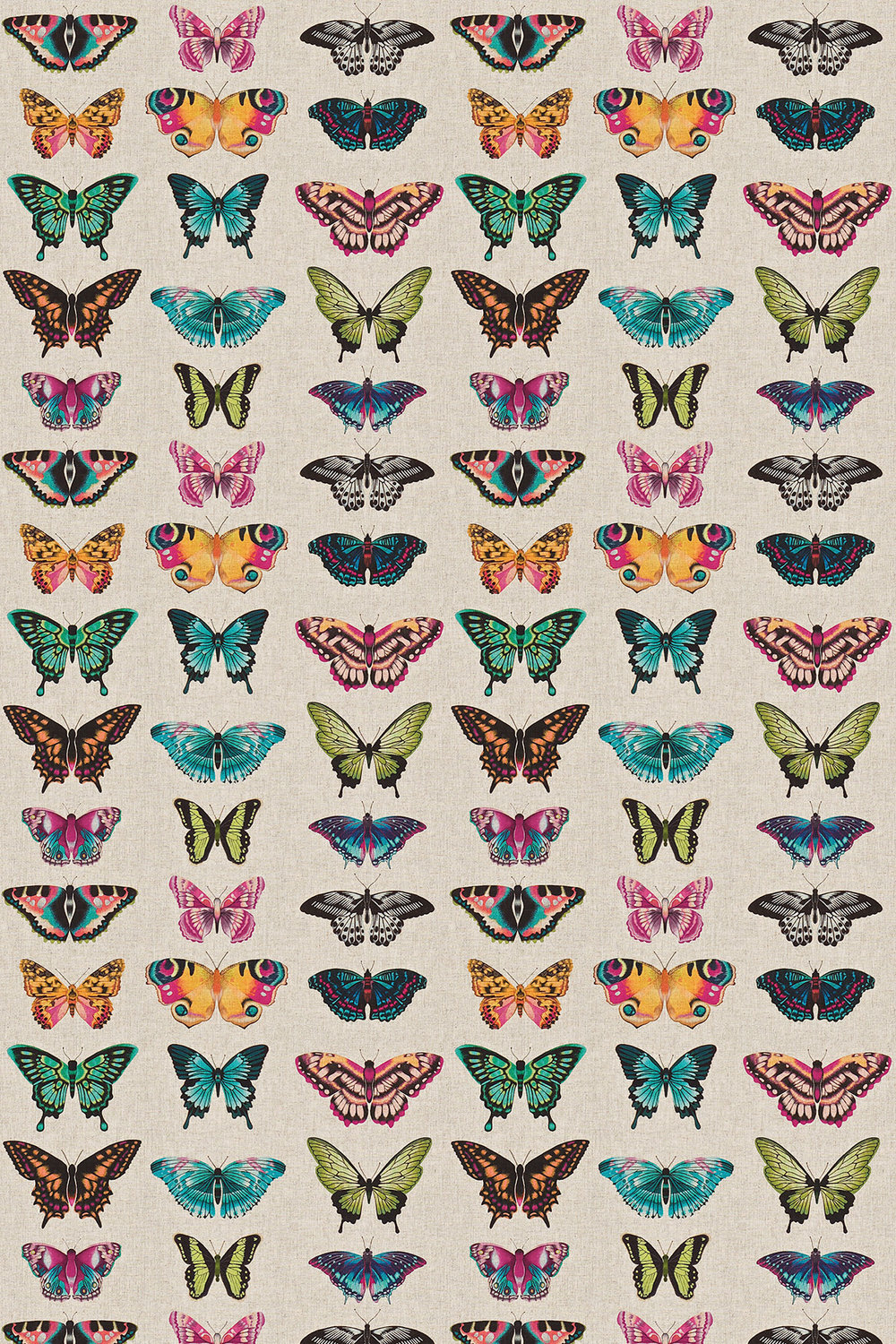The image is a detailed poster featuring an array of butterflies arranged in a repeating pattern against an off-white, slightly textured background. The butterflies are depicted in vivid colors, including shades of blue, pink, green, black, red, orange, yellow, and cream. Each row contains six butterflies that vary in shape and size, but follow a specific repeating order: a multicolored butterfly with pink and blue, followed by a solid pink butterfly, then a black butterfly, and this sequence repeats across and down the entire poster. The butterflies are stylized with noticeable legs and antennae, and their wings showcase a range of patterns and color combinations. The overall effect is a vibrant, orderly display of butterfly diversity on a clean, neutral backdrop.